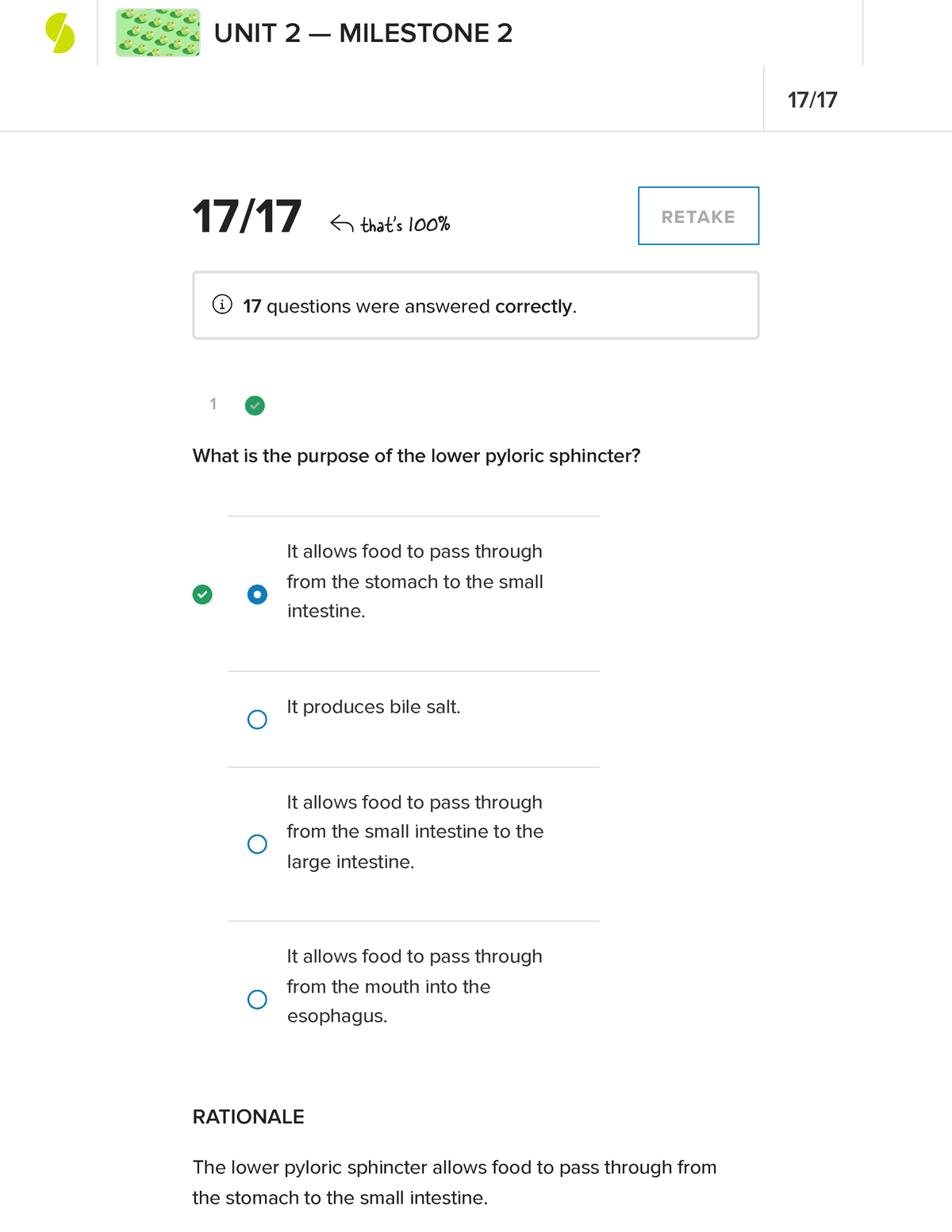**Detailed Caption:**

The image features a predominantly white background. It is divided by a vertical gray line down the middle. On the left side at the top, the text reads "Milestone Two" with two units indicated by dashes. Below this heading, the number "17/17" is displayed alongside the gray line, indicating the total and correct questions answered.

Adjacent to the gray line on the right is another "17/17," confirming that all questions were answered correctly, and accompanied by a notation that this score represents "100%," highlighted with an arrow pointing to it. Just beneath this, there is a white button with the word "Retake" written in gray lettering, encased within a blue border.

Below the scoring section, a detailed question is presented along with multiple-choice answers. The question asks, "What is the purpose of the lower pyloric sphincter?" The chosen correct answer is marked with a green dot and a check mark, stating, "It allows food to pass from the stomach to the small intestine." 

Other answer options are listed as follows:
1. "Produces bile salts" — marked by a circle with a blue outline.
2. "Allows food to pass from the small intestines to the large intestines" — indicated by a standard circle.
3. "Allows food to pass through from the mouth into the esophagus" — also marked by a standard circle.

At the bottom, an explanatory rationale is provided: "The lower pyloric sphincter allows food to pass through the stomach to the small intestine."

The image prominently features the following colors: white, green, several shades of green, black, gray, and blue.